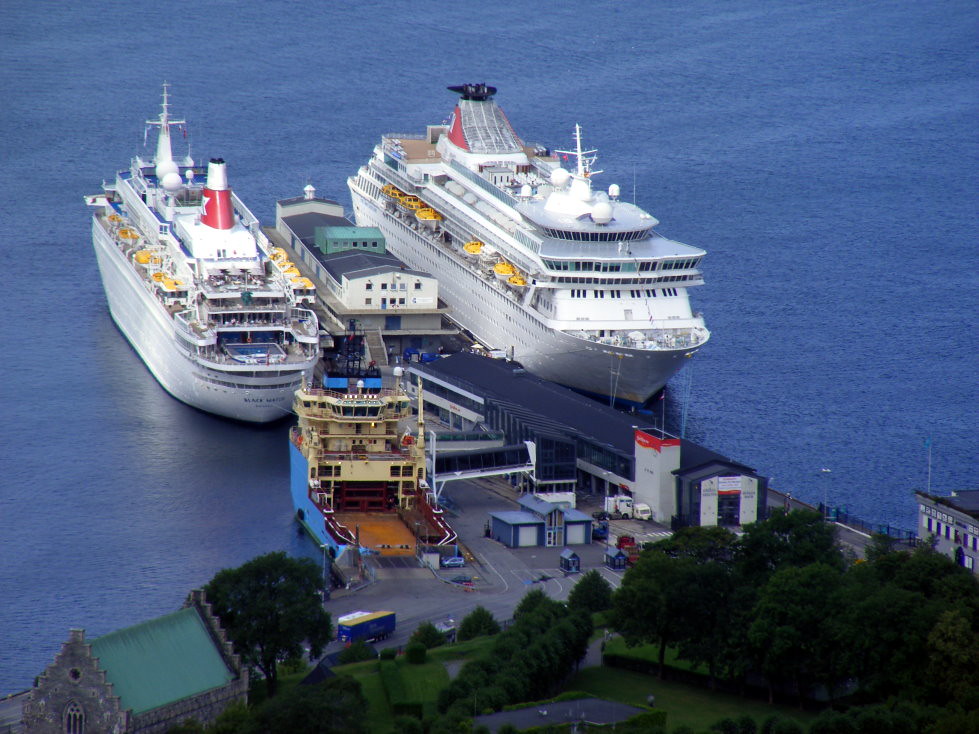This aerial photograph captures a bustling European dock with three distinct ships moored along a picturesque, calm blue waterway. Two massive white ships, potentially cruise liners, are prominently positioned on either side of a dock building. The ship to the right, as viewed from above, is the largest, possibly a luxury liner, and features a significant walkway and checkpoint area for passengers to embark and disembark. On the left, the slightly smaller white ship is marked by a striking red smokestack and similarly busy with passenger activity on its middle deck. Nestled between these giants is a smaller blue vessel, likely a cargo or fishing boat, with its lower deck open and seemingly designed for moving small cargo. In the periphery, a charming European-style building and a lush copse of trees add a touch of antiquity and natural beauty, enhancing the scenic charm of the dock.